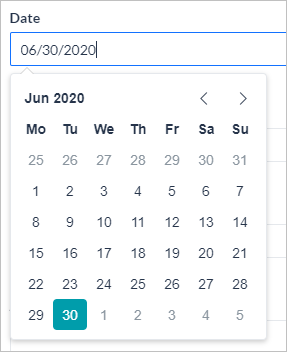This screenshot captures a comprehensive view of a calendar app for June 2020. The calendar's background is white, with black text prominently displaying the dates and days of the week. The calendar begins on May 25th—a Monday—as shown at the top, and proceeds with the remaining days of May (26th through 31st) before transitioning into June. Each day of the week is labeled: Monday, Tuesday, Wednesday, Thursday, Friday, Saturday, and Sunday, respectively.

June 2020 is organized in a 5x7 grid layout starting with Monday, the 1st, and ending on Tuesday, the 30th. The 30th of June is distinctly marked with a green square, highlighting the date in white at its center. Following June, the first day of July 2020 is noted as a Wednesday, with the subsequent dates also included up to Sunday, July 5th. 

The screenshot is devoid of any photographic elements, focusing solely on the clear textual layout and minimalist design of the calendar interface.